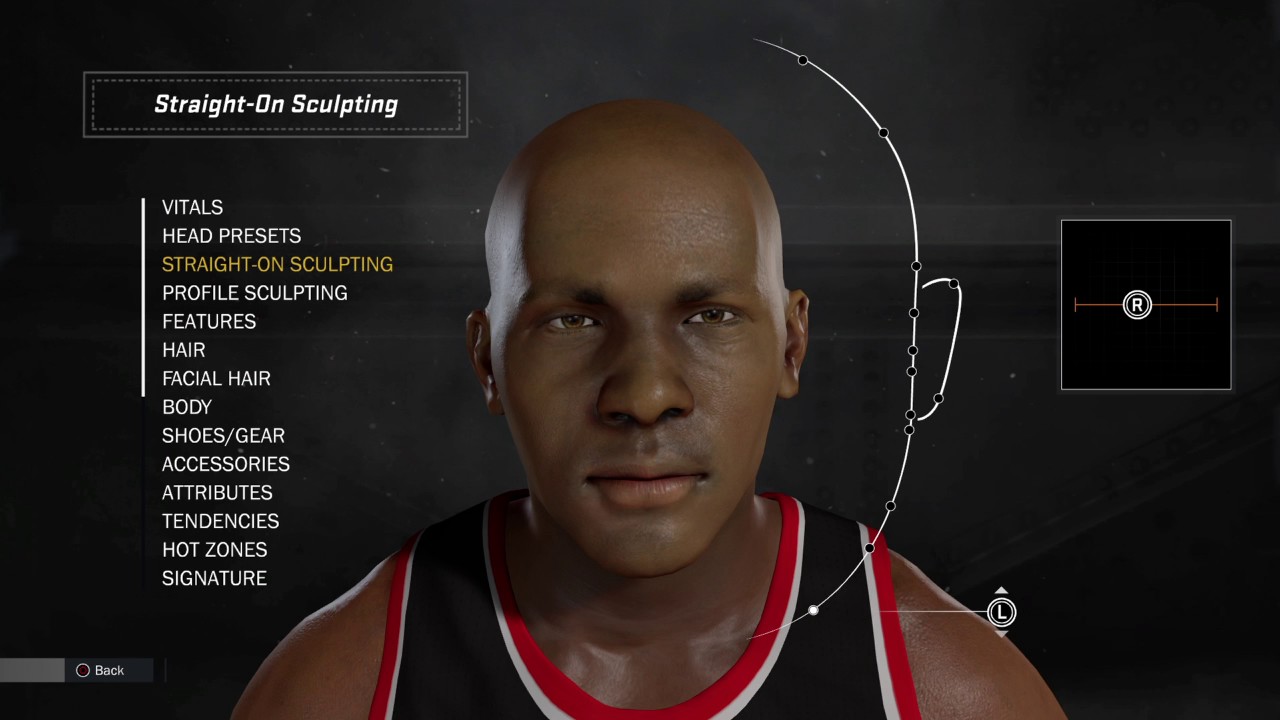The image features a man's face centered against a black background. He appears to be wearing a black basketball jersey with red and white trim. The screen displays various interface options related to character customization, specifically for face sculpting. Highlighted text reads "straight on sculpting" with a detailed list beneath it, including options such as vitals, head presets, profile sculpting, features, hair, facial hair, body, shoes, gear, accessories, attributes, tendencies, hot zones, and signatures.

Next to the man's face, there is an outline diagram of a face with various clickable points, including an ear. To the right of this diagram is a square with the letter "R" inside a circle and a slider that allows you to move the "R" back and forth. Below this, there is a circle with the letter "L" and vertical arrows for up and down adjustments. In the bottom left corner, the screen features a gray bar with a circular button labeled "back." The interface seems to be part of a face sculpting or character creation tool, providing comprehensive customization options for the man's appearance.